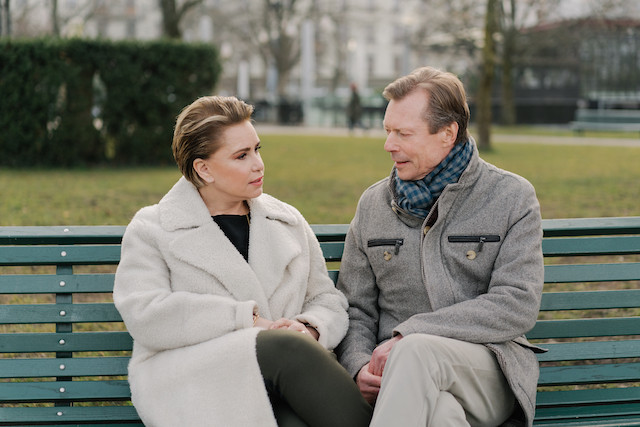Two individuals, a man and a woman, sit closely together on a dark green wooden park bench. The woman, positioned on the left side of the bench, has short brown hair with blonde highlights tucked behind her right ear, revealing her post earrings and eye makeup that accentuates her long eyelashes. She wears a fuzzy, off-white coat over a black top and black pants. Her arms are crossed with her hands resting in her lap, and she slightly turns her head to the right toward the man beside her. The man on the right, with short blondish-brown hair, dons a blue and light green checkered scarf and a gray coat featuring two black-outlined zipper pockets. He wears khaki pants and has his left hand resting on his right hand, which is placed on his lap. The pair, who appear to be between 30 and 50 years old, seem engaged in a conversation, with the woman's expression indicating she is listening intently to the man, who has a serious look on his face. Behind them, a lush park field is visible, with a large green hedge to the left and several spaced trees leading up to an out-of-focus building in the distance.